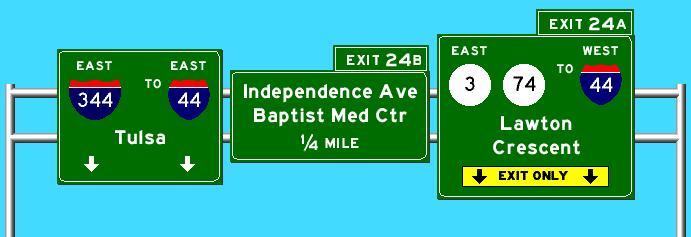This image appears to be computer-generated in a style reminiscent of classic 8-bit video games. The background is a clear, light blue, giving the impression of a cloudless sky. The central focus is on three green traffic signs, typical of those found on interstates or highways, suspended by poles.

The signs are suspended on two main poles positioned on the far left and right, with additional support poles connecting horizontally across the back of the signs. On the leftmost sign, in white lettering, it indicates "East" at the top, followed by "To East Tulsa" with two downward-pointing white arrows. Below this, there are two shield-like icons in red, white, and blue; the left icon displays "344" and the right icon shows "44".

The middle sign consists of two parts. The smaller top sign reads "Exit 24B" in white letters. Beneath it, the larger section reads "Independence Avenue" and "Baptist Medical Center" (abbreviated as "MED CTR"), accompanied by the distance "1/4 mile".

The rightmost sign also has two parts. The upper part displays "Exit 24A" in white letters, followed by "East". Below, two white circles encase black numbers "3" and "74". The word "To" separates these numbers from "West". Additionally, a shield emblem displays "44". Underneath, the text "Lawton Crescent" appears in white, and an elongated yellow rectangle at the bottom reads "Exit Only" in black, flanked by downward-pointing arrows on either side.